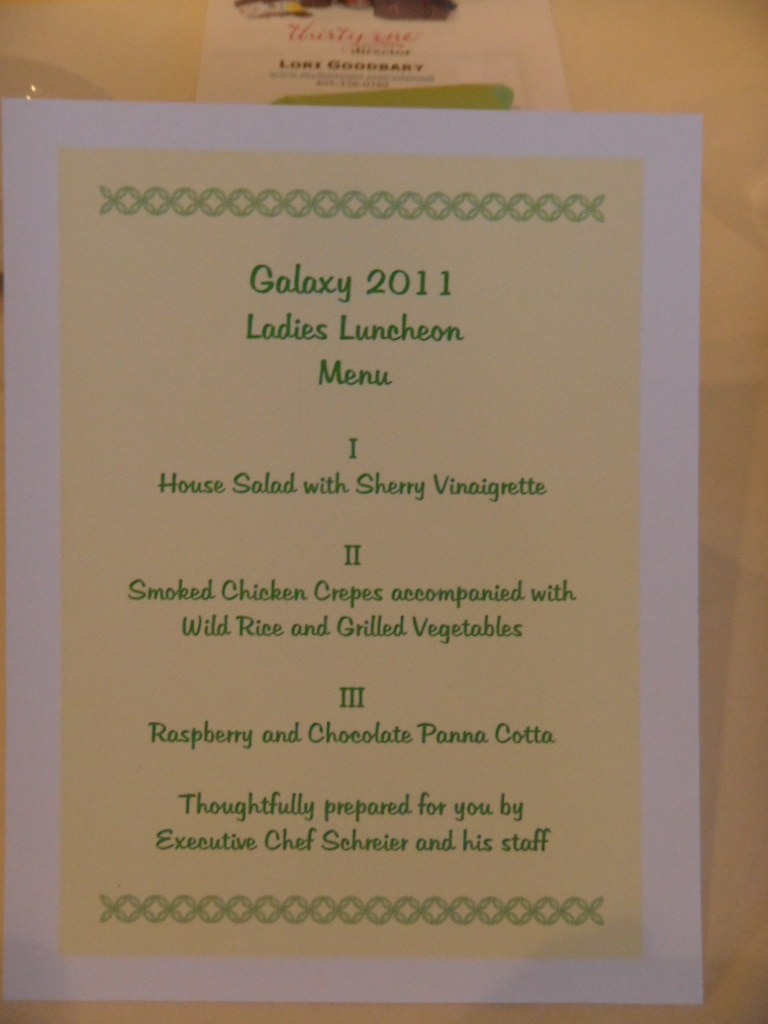A dimly lit photograph showcases a luncheon menu card with distinct white borders and a beige center. The poorly illuminated image suggests it was likely taken indoors with suboptimal lighting conditions. The menu card features a green decorative border at the top, with green lettering that reads, "Galaxy 2011 Latest Luncheon Menu." Below, the menu lists three gourmet offerings: 

1. House Salad with Sherry Vinaigrette
2. Smoked Chicken Crepes Accompanied with Wild Rice and Grilled Vegetables
3. Raspberry and Chocolate Panna Cotta Thoughtfully Prepared for You by Executive Chef Schreier and His Staff

At the bottom of the card, a blue circular design is faintly visible. The card itself appears to be placed on a beige or wooden table, which is blurred and not well-defined due to the poor lighting quality of the photograph.